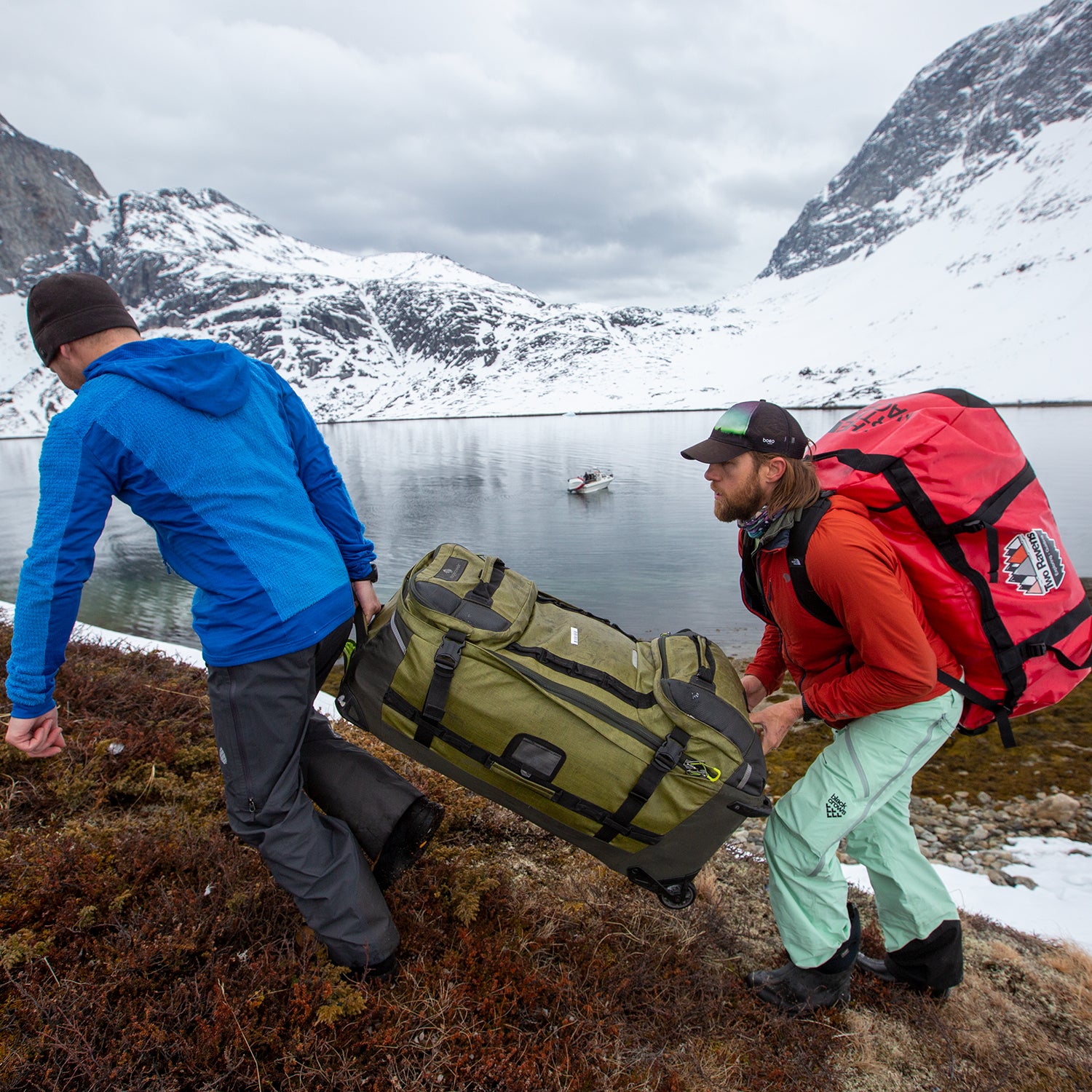Amidst a snowy mountain landscape with white and gray clouds dominating the sky, two Caucasian hikers are captured climbing a small hill. The scene, set in what appears to be freezing conditions, shows the hikers carrying a sizable army green carry-on with black straps between them. The man in front sports a black ski cap, a sweatshirt in two shades of blue (light and dark), gray pants, and black ski pants and shoes. Meanwhile, the man behind him wears a black baseball cap, an orange sweater, teal or light blue cargo pants, and black boots, along with a large red backpack. They seem to be ascending the bare ground, with patches of snow visible both behind them and across a blue-gray lake. A white boat floats on the lake, suggesting a possible mode of arrival or departure for the hikers.